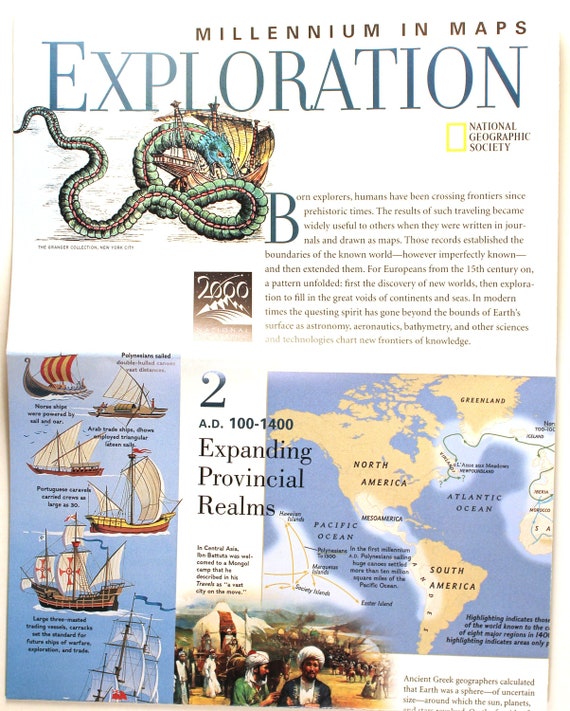The image appears to be a detailed page from a National Geographic magazine, titled "Millennium in Maps: Exploration." At the top, in black letters, it reads "Millennium in Maps," with the word "Exploration" prominently displayed in large blue letters below it. The title is accompanied by the National Geographic Society's logo and a yellow rectangle beside it.

Beneath the title, there's a vivid illustration of a sea serpent attacking a small ship, positioned near the central left of the page. Directly to the right of this illustration, there is a column of text, starting with a large 'B,' though the rest of the text is too small to discern clearly. Underneath the sea serpent illustration, there is a rectangular box with a logo that includes the number '2000' and an image of mountains.

The bottom half of the page is divided into sections. To the left, there's a blue background featuring six illustrations of different ships, each accompanied by small black text. One ship extends off the top of the blue section, while another goes off the bottom. In the center of the page, there is a bold black number '2,' and the text "AD 100-1400 Expanding Provincial Realms."

To the right, there's a map depicting the Atlantic Ocean, with partial views of North America, South America, and Greenland. The map includes labels for the Pacific and Atlantic Oceans, North and South America, and Greenland. Several lines of small black print are scattered throughout the page.

At the bottom middle of the page, there is an image of people with tents, horses, and a crowd in the background against a backdrop of large hills. Additional small black text is found in the bottom right-hand corner of the page.